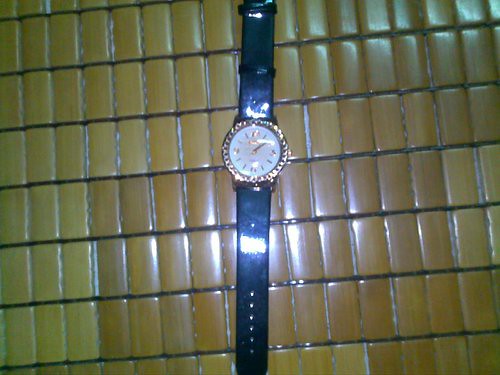This is a detailed color photograph capturing an analog watch positioned on a tiled surface. The tiles, being very small, display a variety of colors including light beige, medium beige, and mustard yellow, creating a visually interesting background. The watch's band is a striking royal blue, reflecting the abundant light in the scene, which produces some glare and masking the exact material; it could be vinyl, plastic, or possibly leather. The watch itself features a gold-tone metal rim, with a white face adorned with Roman numerals, minute, and hour hands all in gold. The interplay of the watch's colors against the tiled surface adds a rich depth to the photograph.